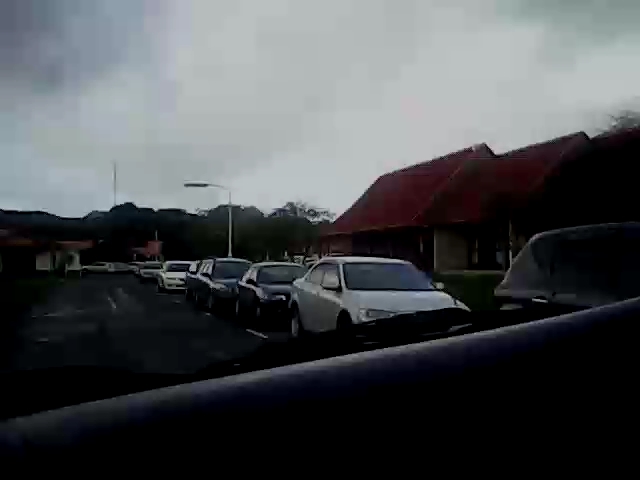An overcast sky filled with heavy gray clouds blankets a residential neighborhood in this photograph, taken from inside a vehicle. The street, lined with closely parked cars, stretches into the distance. The sequence of vehicles includes a black hatchback or SUV followed by a white sedan, another black sedan, yet another black sedan, a white sedan, and then another white sedan, with this pattern continuing down the road. In the backdrop, a house with a distinguishable red roof stands slightly blurred. Surrounding this scene, trees and shrubbery are visible, alongside a streetlight. Additional parked cars, buildings, and signage can also be seen, accompanied by a pole that might belong to a cell phone or radio tower.